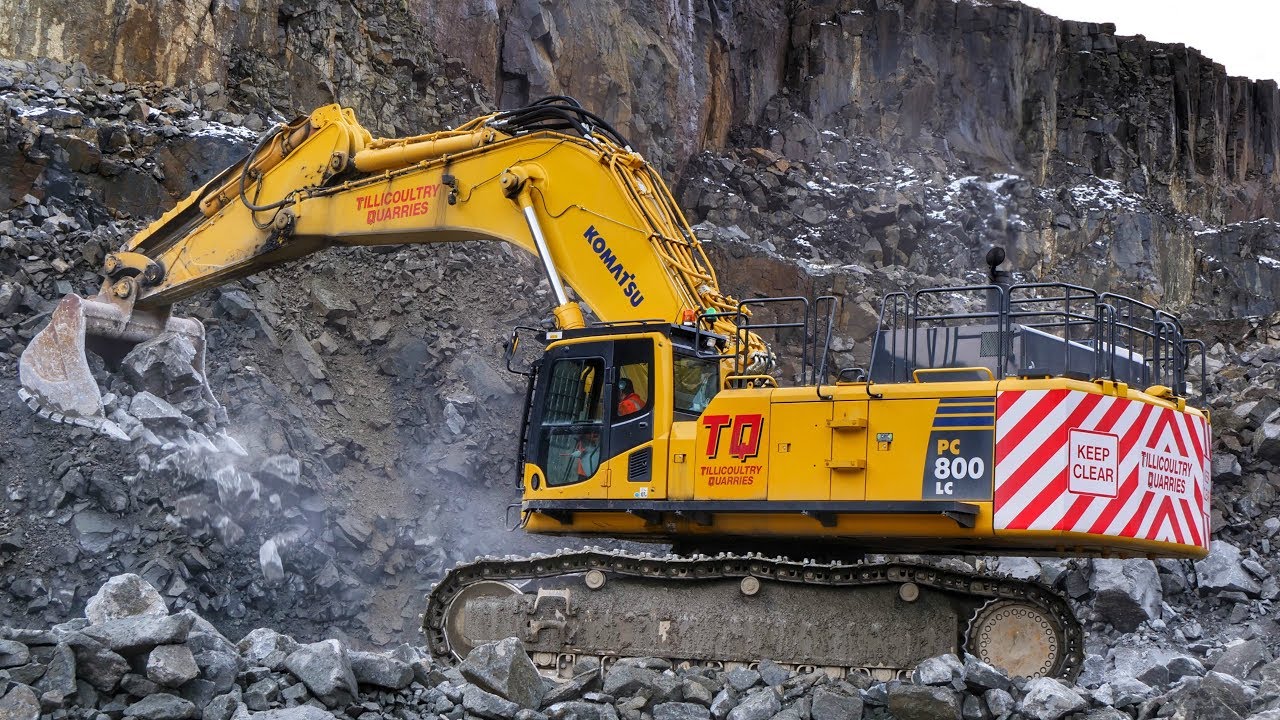The photograph depicts a yellow Komatsu excavator, specifically a PC800LC model, operating in a rock quarry. The machine features a large arm designed for digging and lifting heavy rocks, indicating its robust capability to handle rough terrain with its thick, heavy wheels. The excavator is actively scooping up rocks, potentially granite, from the quarry. The driver's seat is occupied by a worker dressed in an orange outfit and a black protective hat. Notable markings include the text "PC800LC" in yellow and white letters on the side, and the brand name "Komatsu" in blue. The back of the excavator carries a safety warning with "Keep Clear" and "Tilkotree Quarries" in red text, accompanied by red and white striped patterns, alerting onlookers to maintain a safe distance. The scene captures the machinery in action amidst a rugged, rocky backdrop.